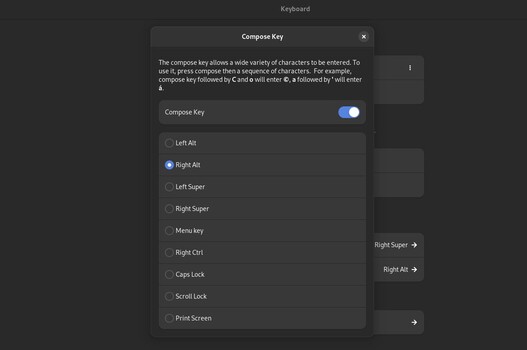The image is a screenshot taken from a tablet or mobile device, featuring an application with a sleek, dark-themed User Interface (UI). The app has a black background with buttons and UI elements in various shades of gray, while the text is prominently displayed in white for high contrast and readability.

At the top of the screen, the title reads "Keyboard," indicating the section of the settings being viewed. Below the title, an open window titled "Compose Key" provides information about this feature. The descriptive text explains: "The Compose Key allows a wide variety of characters to be entered. To use it, press Compose, then a sequence of characters. For example, Compose Key followed by C and O will enter a specific character."

The Compose Key feature is currently activated. Several options are available for assigning the Compose Key function, such as Left Alt, Right Alt, Left Super, Right Super, Menu Key, Right Control, Caps Lock, Scroll Lock, and Print Screen. Among these, the Right Alt key is selected, making it the designated Compose Key. This selection is highlighted, while the other options remain unselected and are displayed against a gray background.